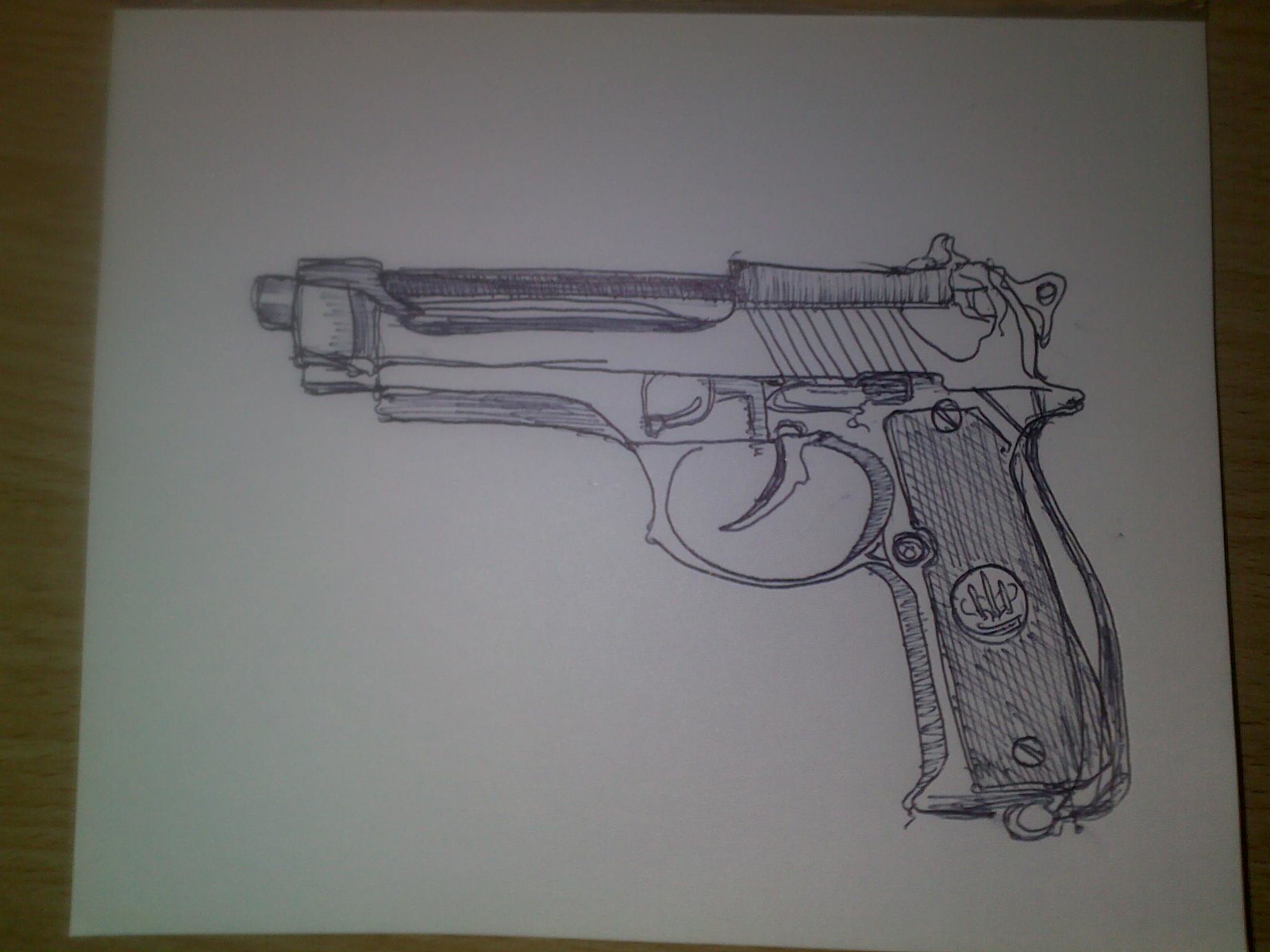A meticulously detailed pen drawing of a 9mm or Airsoft handgun is depicted on a piece of white printer paper in landscape orientation. The artwork features an intricate outline as though the artist traced over a photograph, capturing every ridge and groove of the firearm. The discernable elements include the short muzzle, the visible trigger, a safety mechanism, and the hammer at the back in the slide. The grip is distinctly highlighted, showcasing a white plastic inset secured by three screws—notably one at the top, one at the bottom, and one positioned to the left. A prominent logo or emblem, consisting of three upright white pieces accompanied by some text and lines, is also etched into the handle. The paper rests on a light tan desk, set against a backdrop of slightly dim lighting, emphasizing the contrast and details of the pen drawing.